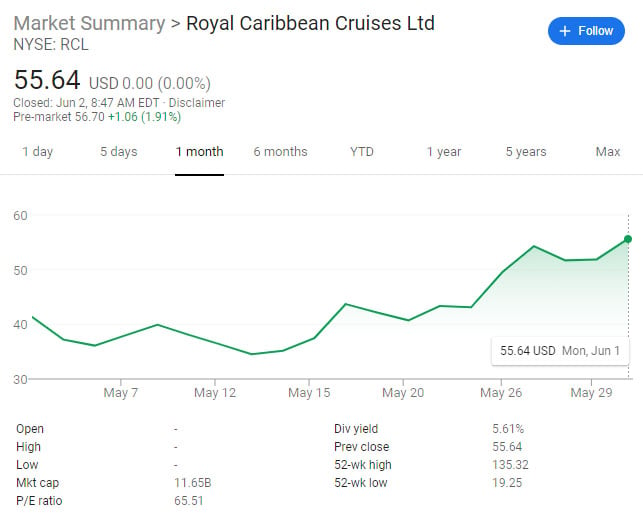This image depicts a market summary page for the stock of Royal Caribbean Cruises, LTD. In the upper left corner of the page, the words "Market Summary" are written in gray font, followed by a forward arrow pointing to the company's name, "Royal Caribbean Cruises, LTD," in black font. The upper right corner features a blue rectangle with rounded edges, containing the word "Follow" in white font along with a white plus sign.

On the left side, we see additional details: "NYSE" (New York Stock Exchange) and the stock symbol "RCL." The current stock price is displayed as $55.64, and it is noted that this price was as of June 2nd at 8:47 a.m. EDT. Below this, a stock chart is visible, with options to view trends over various time periods: one day, five days, one month, six months, year-to-date, one year, five years, or the maximum available. The chart is set to display data for one month, specifically May.

At the bottom of the chart, data for May is shown. The stock price hovered around $40 at the beginning of the month and dipped to approximately $35 around May 13th, before trending upwards. By May 29th, the stock price approached its peak for the month. The line chart is colored green, indicating positive movement. Beneath the chart, there are three columns of additional statistics, providing further insights into the stock's performance. The image lacks any website-specific headers or footers, making it difficult to determine its source.